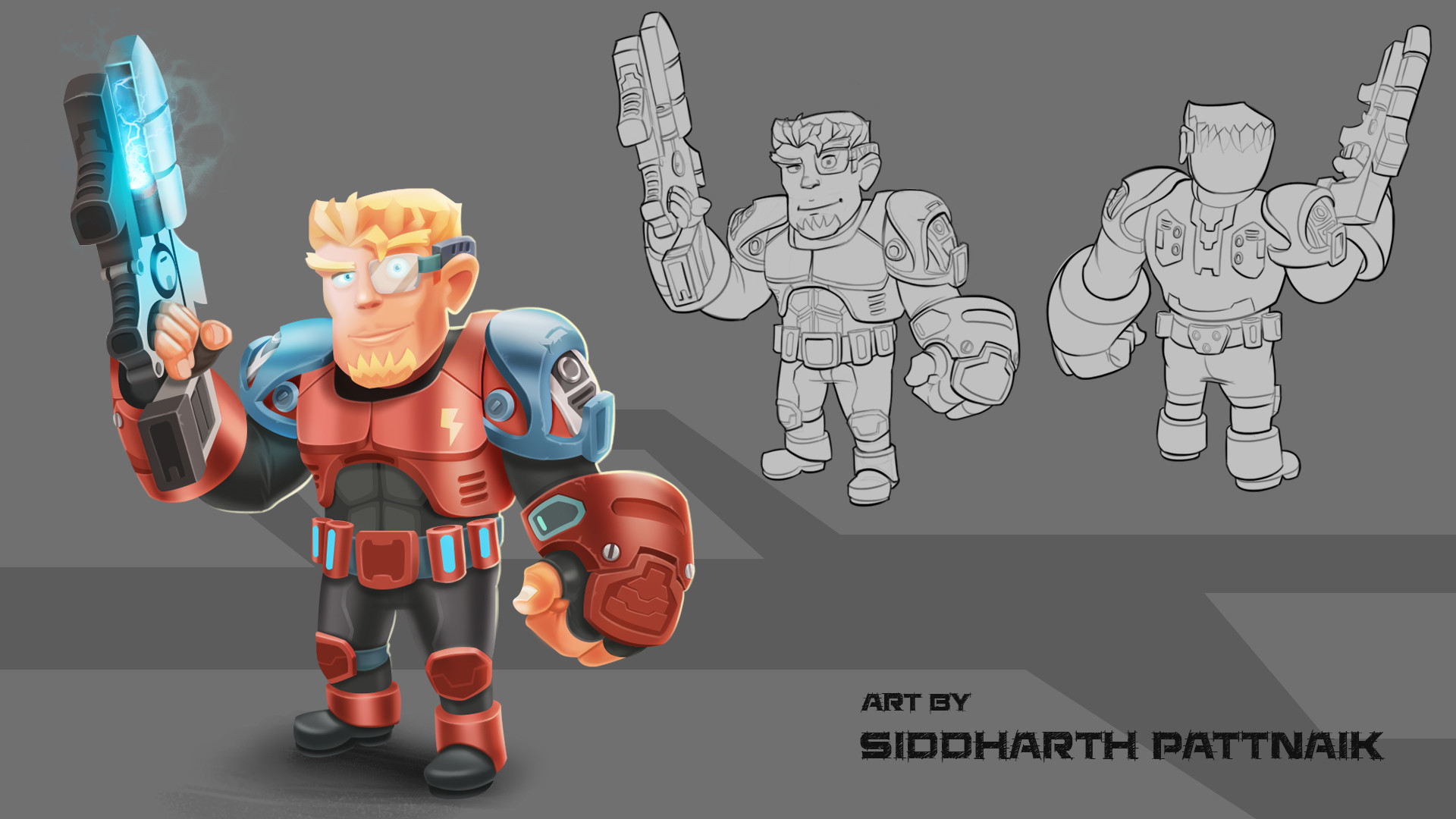This image showcases a character design for a potential mobile game or toy advertisement, drawn by artist Siddharth Patnaik. Set against a gray background with darker gray horizontal lines, the design presents a futuristic soldier with a cartoonish, exaggerated appearance. The primary, colorful depiction on the left features the character in red and blue armor over a black outfit. Notable details include a blonde flat-top haircut, a yellow goatee, and a high-tech monocle-like eyepiece that extends around his ear. The character wields a large gun emitting blue energy, complemented by prominent red gauntlets and blue metal shoulder armor. To the right are two black-and-white sketches, portraying front and back views of the same character, highlighting its multi-perspective design. The text "Art by Siddharth Patnaik" is inscribed in black in the bottom-right corner, emphasizing the artist's contribution. This unified portrayal combines key elements from different perspectives to emphasize the intricate and humorous nature of the character's design.